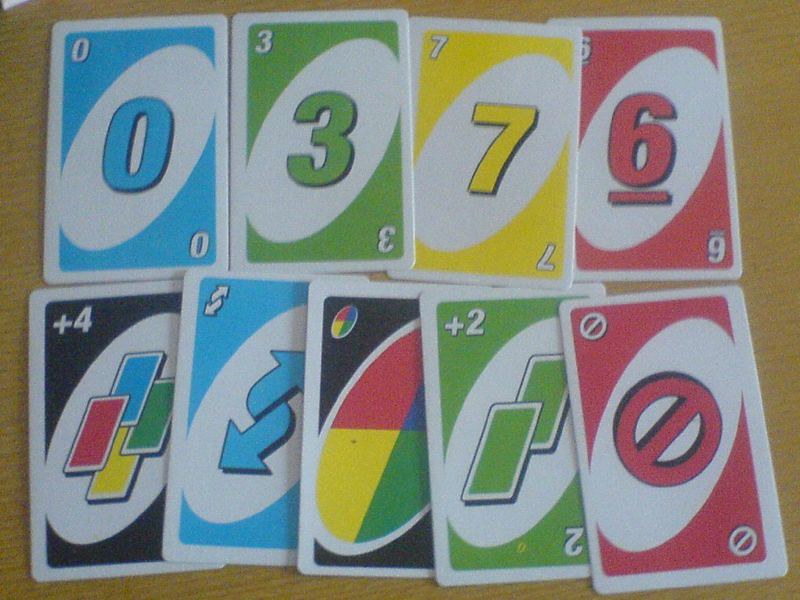This top-down photo showcases eight UNO playing cards neatly arranged in two rows of four on a light beige, wood-grain table. Each card features its respective design and number prominently centered within a white oval that spans diagonally from the bottom left to the upper right, all surrounded by bold black outlines. The numbers are duplicated in the upper left and bottom right corners, rendered in striking white font with black borders for clarity.

In the top row, from left to right, the cards are:
1. A blue '0' card.
2. A green '3' card.
3. A yellow '7' card.
4. A red '6' card, where the number six is underlined in red to distinguish it from a potential nine.

The bottom row features:
1. A 'Wild Draw Four' card displaying four differently colored cards in the center.
2. A 'Reverse' card, signified by two white reversing arrows against a backdrop featuring a four-colored circle.
3. A 'Draw Two' card, indicating the action with a multi-colored plus two symbol.
4. A red 'Skip' card, marked by a red cancel symbol.

This well-organized display clearly illustrates the diversity and vividness inherent to an UNO deck.